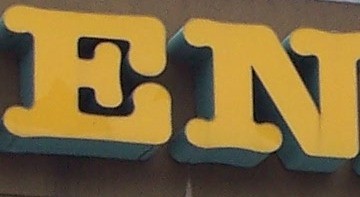This color photograph, taken in landscape mode, captures a cropped portion of a sign on a building with a dark brown background. The image zooms in on two capitalized bubble letters, "E" and "N," rendered in a 3D serif font. Both letters are a bold goldish yellow, with shadowed edges in dark gray, giving them a raised appearance. The letter "N" is slightly clipped on the right-hand side, suggesting a larger sign beyond the photo's borders. There are no other elements in the photo, as it focuses solely on these detailed letters against the brown wall. The image itself is small and wider rather than taller.